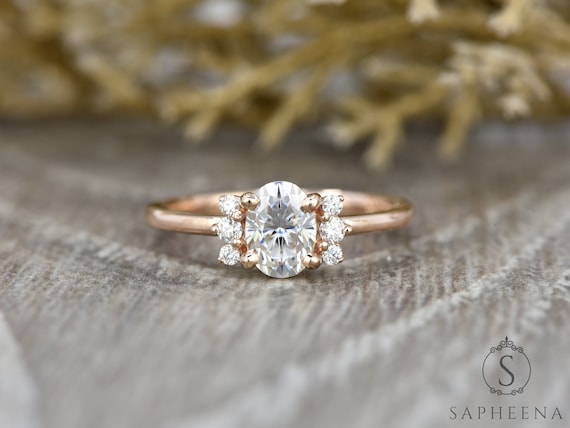This image showcases an elegant engagement ring prominently featuring a large, oval-cut white diamond in the center. The oval diamond is secured by four curved metal posts, adding a touch of sophistication. Flanking the central gem are three smaller diamonds on each side, arranged in a way that they cascade down the band like delicate wings. The band itself is crafted from gold, although it could be perceived as rose gold or a gold-copper alloy. The ring is displayed on what appears to be a gray, stone-like surface, possibly granite, with a blurred background featuring natural elements like tree branches or plants. In the lower right corner, the brand name "Saphena" is elegantly inscribed beside a distinctive logo, comprising an 'S' encircled and adorned with decorative squiggles, marking the prestigious maker of this stunning piece.